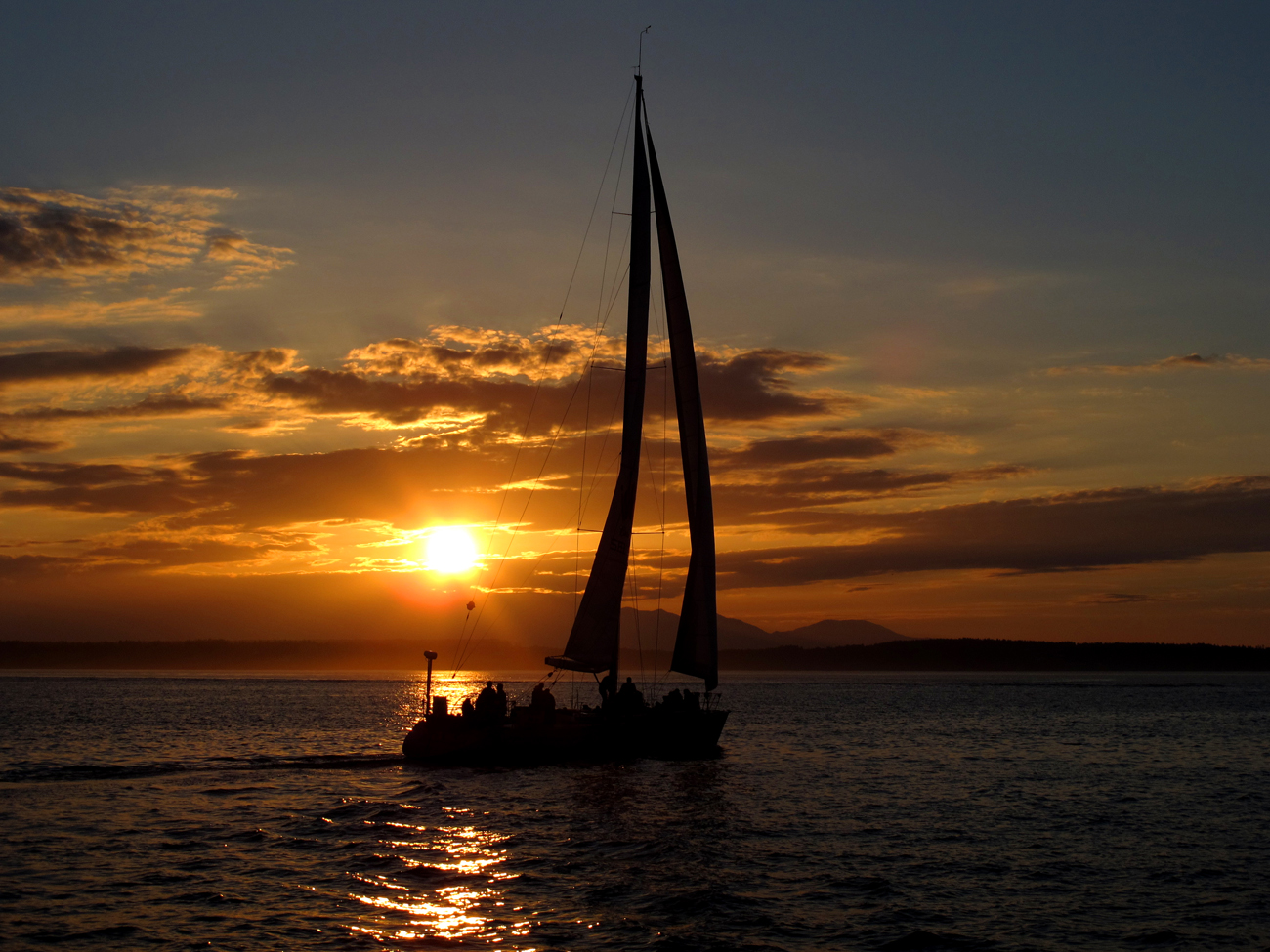The image is a stunning color photograph of a sailboat peacefully gliding across the sea during an evening sunset. The boat, with its two tall sails and thin wires extending upward, is silhouetted against a breathtaking twilight sky. The sky is a beautiful gradient, with the lower portion illuminated by a dark golden light from the setting sun, which reflects across the tranquil sea, while the upper half shifts to a serene purple hue. The silhouette of the sailboat is accentuated by this rich interplay of colors. Dotted along the deck, a number of people are visible on the boat, though their facial details remain indistinct. Far on the horizon, there appears to be a landform or a dense cloud cover, adding depth to the scene. The overall ambiance is one of calm and beauty, capturing the essence of a serene evening at sea.